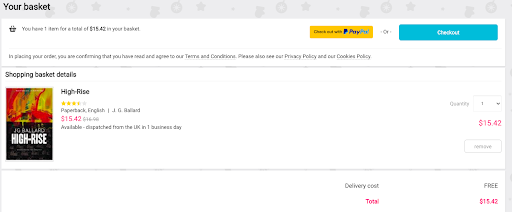Caption:

The image shows a screenshot of an online shopping cart from a website. At the top of the page, there is a grayish bar with the text "Your Basket" in black. Below this, some text and the PayPal logo appear within a yellow box. Beneath that, a blue box labeled "Shopping Basket Details" is visible. The main item featured in the basket appears to be a book. The cover of the book is divided into two parts: the bottom half is black with bold white text reading "High Rise," and the top half is a gradient of red, yellow, and orange. To the right of the book cover, additional details are listed: the book's title "High Rise," a four-star rating, its format as a paperback, and the language as English. The price of the book is displayed as $15.42 in red. Next to this, it states the delivery cost is free. At the bottom of the section, in red text, it shows the total price as $15.42. It appears to be a checkout basket, possibly from Amazon.